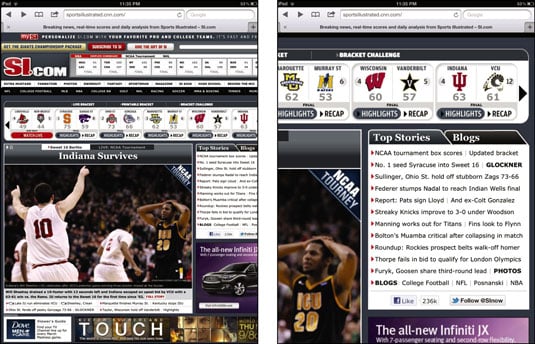**Caption:**

A composite screenshot showcases two distinct views of an SI.com webpage, a now possibly defunct sports website, focused on college basketball updates. The larger view presents the entire webpage, whereas the smaller, more detailed view zooms in on specific elements of the same page.

The webpage's header features the recognizable red SI logo, a red circle, and "COM" in bold letters. Interactive elements such as a URL bar, search icon, navigation arrows, and bookmark options are visible, while a share icon points outward to the right.

The main image captures an intense moment from a college basketball game: players wearing white jerseys with red lettering. A prominent headline reads "Indiana Survives," indicating a victorious outcome for Indiana, probably in a college basketball game, supported by game scores displayed in a top bezel. This bezel lists matchups and scores: Ball State vs. Alabama (49-44, in-progress), Syracuse vs. Kansas State (75-59, final), Ohio State vs. Gonzaga (73-66, final), and Indiana's 63-point score. Vanderbilt vs. Wisconsin is noted, possibly with a 40-57 score in Vanderbilt's favor, as the text states "Recap."

A close-up of the right-hand side showcases a jersey with "ICU" in gold and the number 20, and beneath it, a detailed list of "Top Stories." Highlights include:

- NCAA Tournament Box Scores
- Updated bracket and Syracuse advancing to the Sweet 16
- Recap by Glockner and a commentary on Sullinger aiding Ohio State's victory over Gonzaga
- Federer defeating Nadal in tennis to reach the Indian Wells final
- Report on the Patriots signing Lloyd and ex-Colt Anthony Gonzalez

Other bullet points include:
- NY Knicks' improvement to a 7-3-0 record under Woodson
- Manning's workout for the Titans & potential moves by the Dolphins
- Bolton's Muamba critical after collapsing during a match
- Highlighting Rookies' home run and Thorpe's failed Olympic bid
- Golf update on Furek and Goosen sharing a lead

There's also a "Photos" section, notable for its bold text, followed by blog categories such as College Football, NFL, and NBA lines, and a blurred mention of Posnanski. Social media details show 236k likes on Facebook and a follow suggestion for "SHOW" on Twitter, likely associated with Brian Shaw. 

The detailed layout serves sports enthusiasts by providing a comprehensive snapshot of current sports events, scores, and news stories.